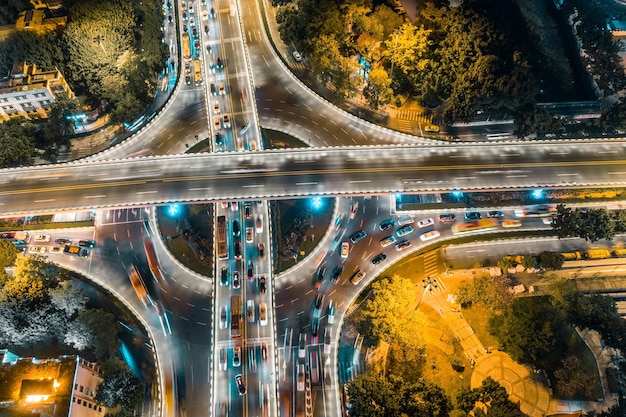The overhead drone photo, likely taken at nighttime, captures a bustling urban scene with a prominent highway and expressway intersection forming a cross shape over a large roundabout. The image reveals heavy traffic with some cars at a standstill and others moving rapidly, leaving trails of light that create a sense of motion. The area is lit by yellowish-gold street lamps, enhancing the night-time setting. On the left and right sides of the image, numerous buildings and city blocks are visible, while a park area occupies the bottom right corner. Additional greenery and trees can be seen interspersed throughout the cityscape, particularly in the top right section. The use of blue lights lining the edge of the upper roads further highlights the vibrant, busy atmosphere of this urban landscape.